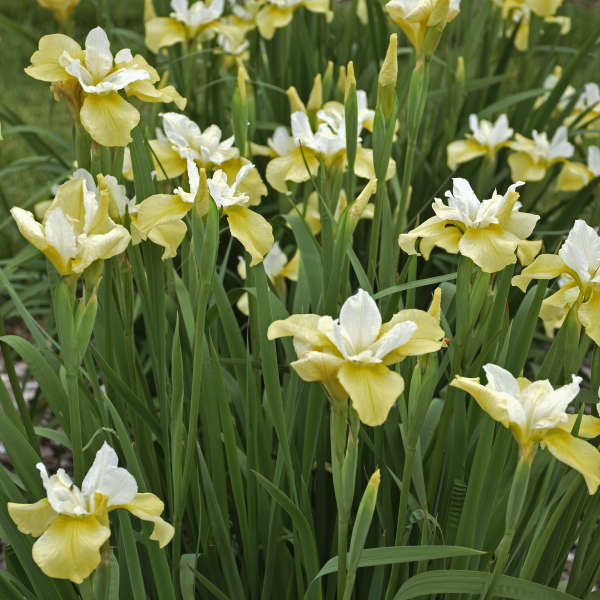This photograph, possibly captured under sunny conditions, features a vivid patch of yellow flowers with intricate details that suggest professional quality. The image is densely populated, stretching from top to bottom and left to right with about 15 prominent flowers. Each flower displays two sets of petals: the outer ones are long and yellow, enveloping a smaller, inner group of white petals. There are also multiple unopened buds, showing green enclosures with yellow tips, indicating future blooms. The foreground and background are dominated by long green stems and slender leaves, with occasional brown elements that are indistinguishable. The lush greenery and the bloom of flowers create a cohesive and immersive botanical scene. No identifying text or labels are present in the picture.